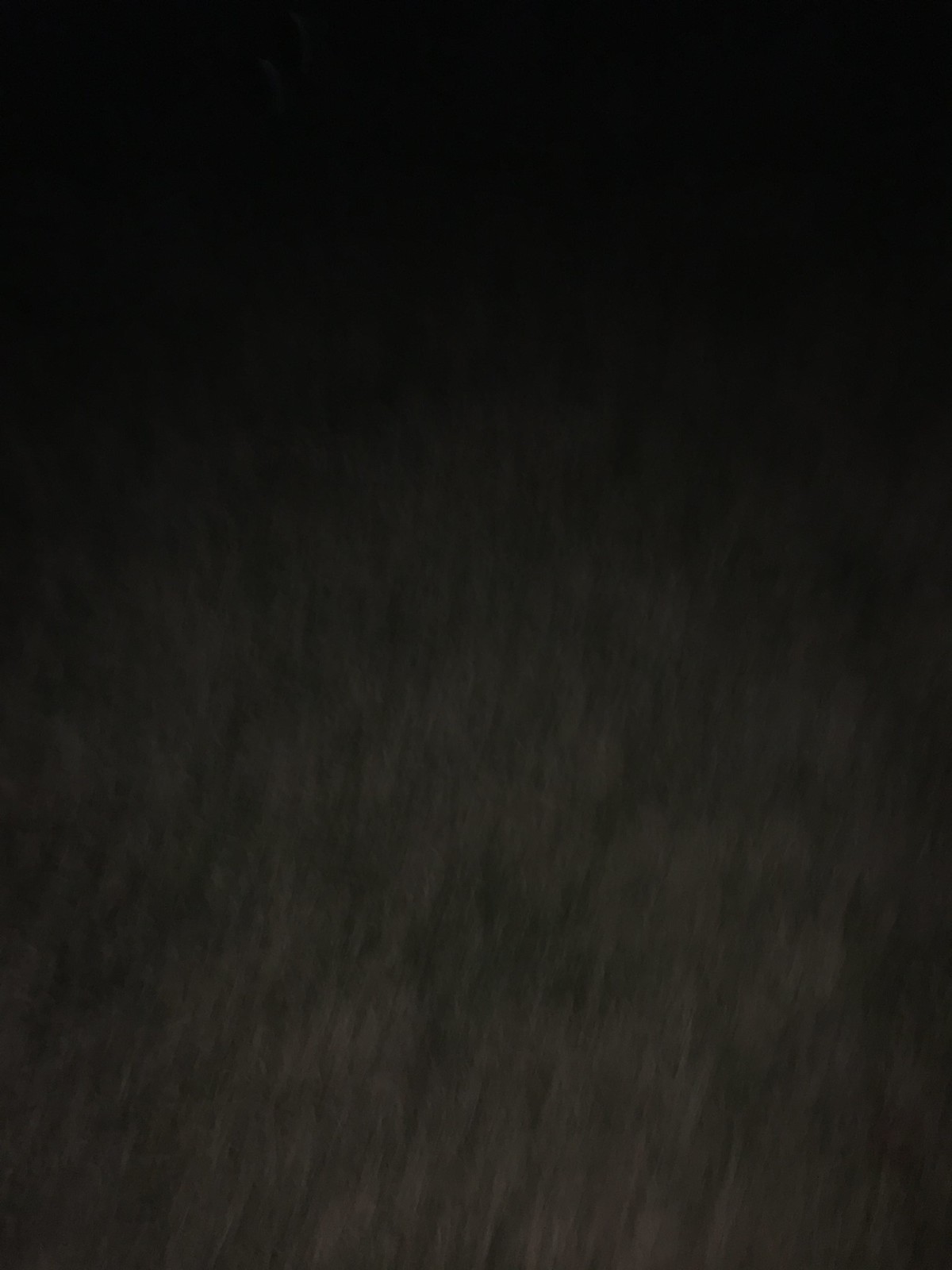The image is a heavily blurred photograph with a dark blackish-gray background, possibly taken at night. It appears to be a rectangular shape, longer in length than width, with some indication of depth through a gradient of colors. The top portion of the image is almost entirely black, punctuated by two tiny white smudges. As you move downwards, a subtle gradient emerges, transitioning from black to lighter gray, with tiny black spots interspersed. The overall effect indicates motion blur, potentially from a head camera, with some fisheye distortion around the edges. The blurred texture and color suggest it might be a close-up of an animal's fur or carpet fibers, but the exact material remains unclear. Despite the blurriness, faint textural elements are visible, primarily near the bottom two-thirds of the image.